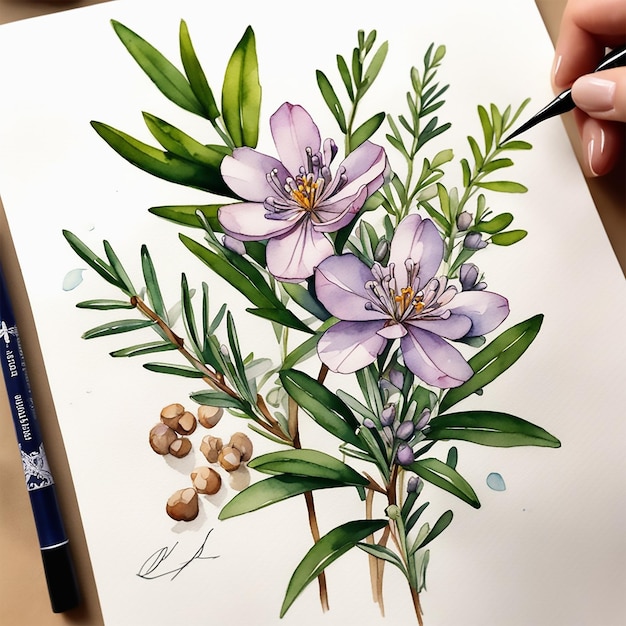The image captures a detailed drawing of two light lavender-colored orchids on a white piece of paper, set against a beige-colored surface. A woman's hand, with neatly beige-painted nails, is positioned at the top right corner, holding a black pen or marker as she delicately works on the artwork. The orchids, surrounded by uniformly pointed almond-shaped green leaves, are accompanied by a few small elements that resemble walnuts on the lower left side of the composition. Below these elements, there's a signature, presumably from the artist. To the left side of the paper, there is a blue pen with white writing, capped and resting on the surface. The drawing is centrally positioned but slightly angled to the left, with the entire scene suggesting an intimate, creative moment in progress.